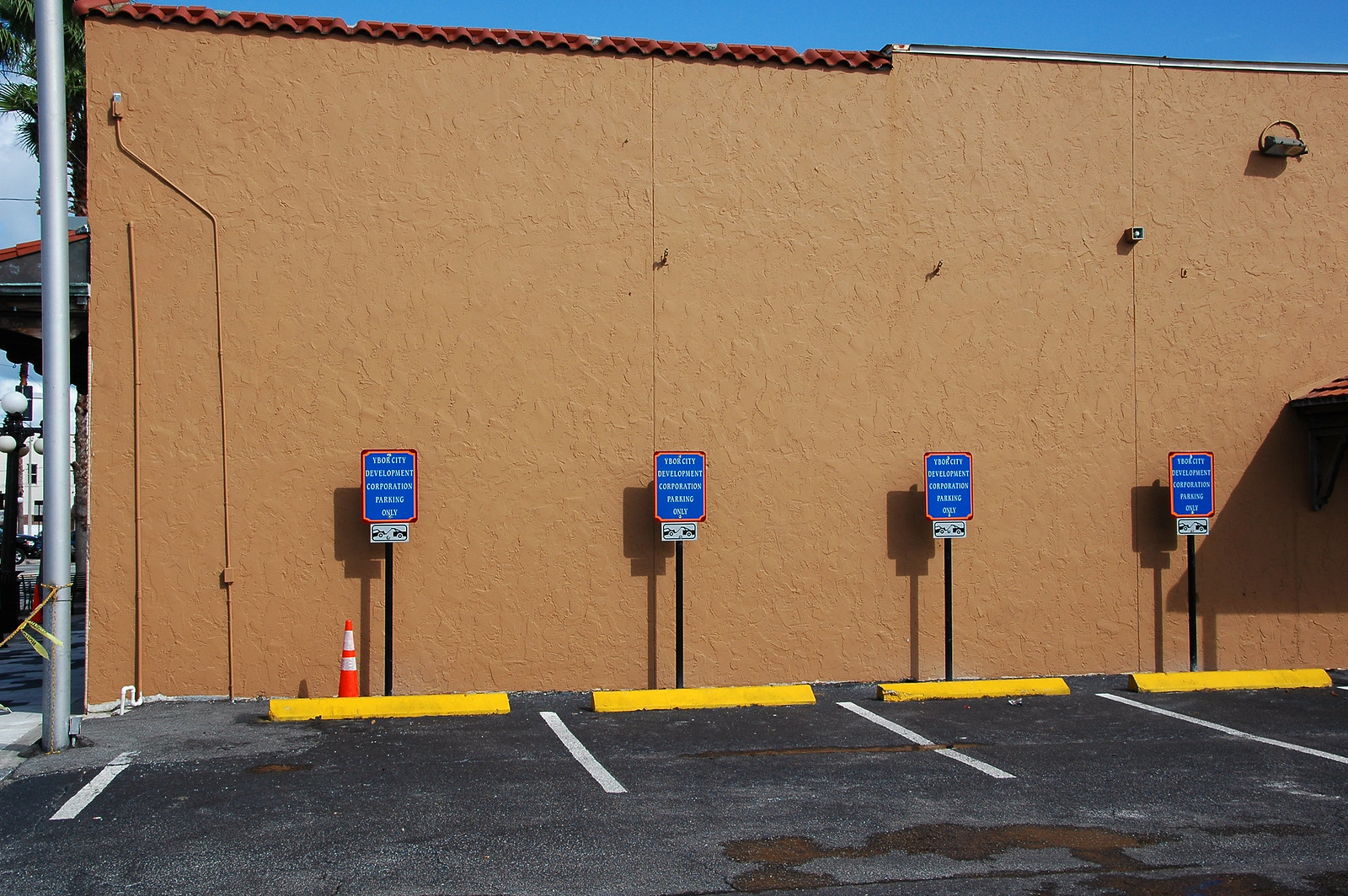The image portrays the side of a tan-colored commercial building, possibly stucco or plastered concrete, with a red, wavy tin roof partially visible along the top. The building has a flat roofline with some red shingles, similar to those seen on Mexican restaurants, and an awning on the left hinting that it might be a restaurant. The scene includes a black asphalt parking lot with four distinct parking spaces, demarcated by white lines and terminated by yellow parking stops. Each parking space is marked by a blue sign with a red border mounted on a black post, indicating specialized parking such as city development corporation parking, with an accompanying image of a car being towed. There is a noticeable orange traffic cone with white stripes positioned by the leftmost sign. The background features a bright blue sky and hints of a city street and sidewalk on the far left, alongside a street lamp. Additionally, surveillance cameras are mounted on the building, overseeing the parking area.